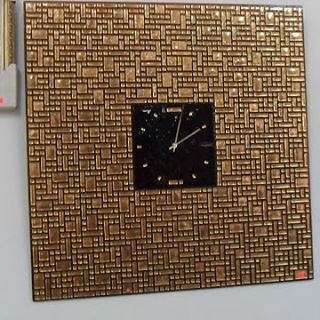This image features a distinctive wall clock centered against a white background. The clock itself has a small, black face, adorned with gold hands and minimalistic gold line markers in place of traditional numbers. Notably, the 12 o'clock and 6 o'clock positions are highlighted with white rectangular backgrounds. Surrounding the clock face is a large, square brown frame that appears to have a basket weave pattern, suggesting it is carved out of wood and then stained and polished for a refined finish. The frame is consistent in width on all sides, creating a striking contrast against the white wall it hangs on. It is precisely two minutes past two o'clock.